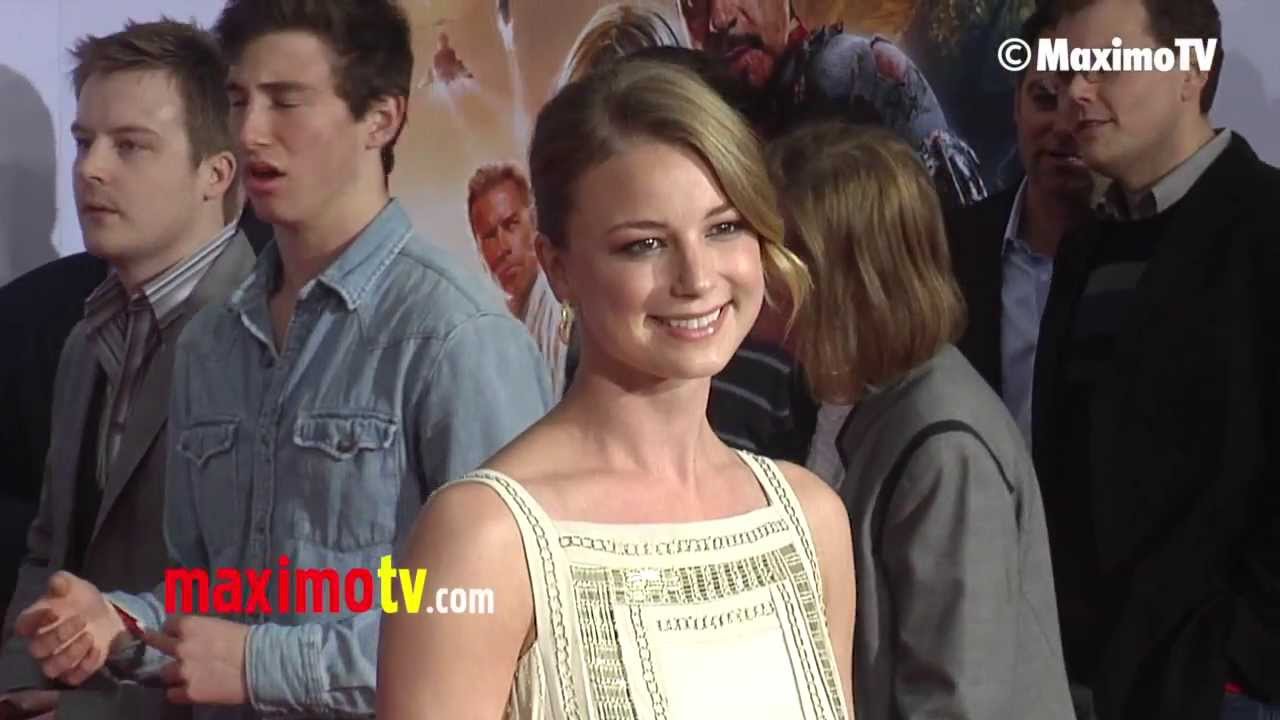This image captures a nighttime scene at a movie premiere, likely for a Marvel or Iron Man film. The central figure is a female actress with blonde hair and light skin, smiling and posing for press or journalists on what appears to be a red carpet. Her hair is styled in a ponytail with curled bangs framing her face. She is dressed in a beige, sleeveless tank top adorned with light green decorations. 

Behind her, to the left, two men of Caucasian descent are visible, walking or looking towards the left. More people are crowding around on the right-hand side, although their faces aren't clearly visible. The backdrop features a movie poster depicting at least two male figures and a helicopter, suggesting action content.

Text elements include a white copyright symbol followed by 'Maximo TV' in the upper right-hand corner, and another logo at the bottom left with 'Maximo' in red, 'TV' in yellow, and '.com' in white.